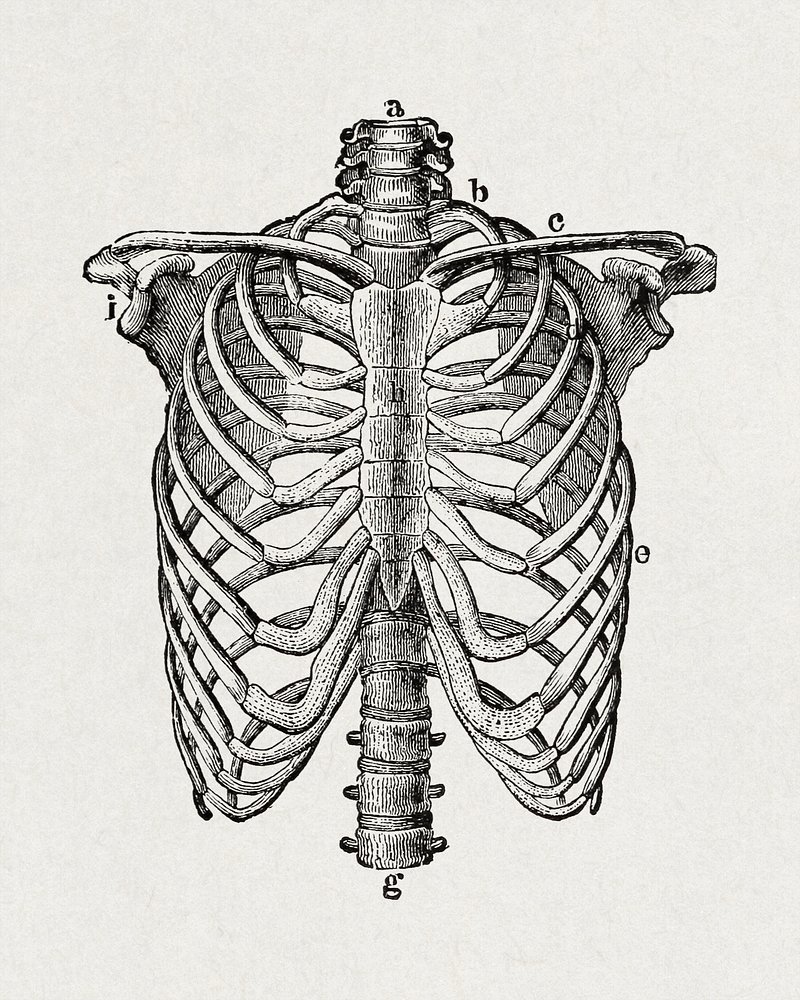In this detailed hand-drawn black and white diagram of the human torso, the artwork meticulously illustrates the spine and ribcage with anatomical precision. The drawing focuses solely on the skeletal structure, from the neck down to the lower spine, with the entire composition set against a grayish off-white background typical of aged paper.

The spine is prominently featured, marked with several letters that seem to reference specific points in the anatomy. At the top of the spine, where the neck bones terminate, the letter "A" is inscribed in an old typewriter-style font. Following down to where the neck meets the shoulders, the letter "B" appears. Over the right clavicle, "C" is noted, while the letter "E" is situated on the ribcage. The bottom of the spinal column bears the letter "G."

Additionally, the shoulder blade area on the left side is labelled "J," and within the ribcage, on the sternum, the letter "H" can be found. Each bone is drawn with thin, precise black lines that add depth and convey the intricacies of human anatomy, indicative of the artist's thorough understanding of the subject. The background remains completely blank apart from these annotations, emphasizing the clarity of the skeletal representation without any distractions. 

This intricate and thoughtfully detailed drawing effectively showcases the main anatomical features of the torso, making it a valuable visual aid for studying the human skeleton.